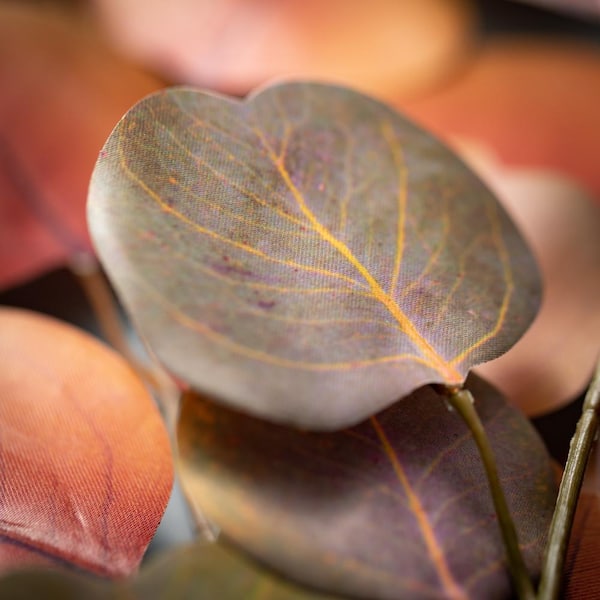This close-up photo captures a fake plant composed of plastic stems and fibrous plastic leaves. The plant features leaves in two distinct shades: a reddish fall hue and a brownish color, resembling dried and dying foliage. The stems are brown, while the leaves have bright yellow veins running through them. The scene is detailed, showing a leaf with pronounced yellow lines and a brownish golden tan shade. There are two stems on the right-hand side, with a leaf extending below and another leaf rising above it. Additional leaves appear slightly out of focus, with some looking darker green with yellow veins and others looking more reddish without evident veins. The background is blurred, highlighting the leaves, and a blurred hand with a distinguishable thumb is visible on the left side. There is no text in the photo.